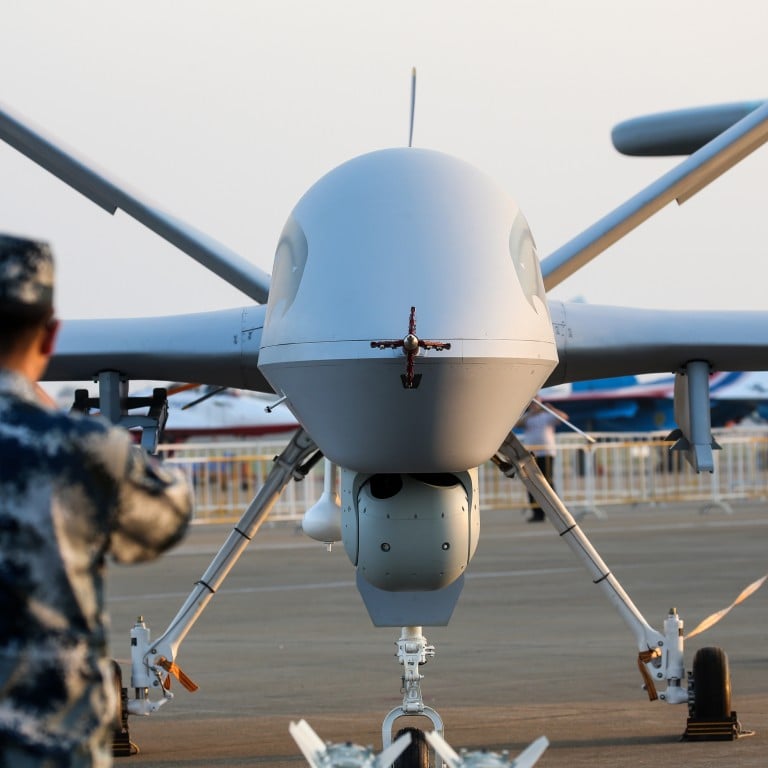This photograph depicts a gray military drone centrally positioned on a military base, with a soldier in tan and black camouflage uniform standing in front of it. The drone, about the size of a Prius or half the size of a small Cessna airplane, has a body with front and rear wheels, a rear wing, and two diagonal poles attached to a satellite dish-like apparatus. The drone rests on blocks and has a tether line on its right rear wheel. In the background, there are additional military personnel, a plane, some railings, and a clear sky, enhancing the scene's depth. The overall color palette includes various shades of gray, white, blue, red, and black, with the fence in the background being white. This detailed setting underscores the organized and technical environment of a military base.